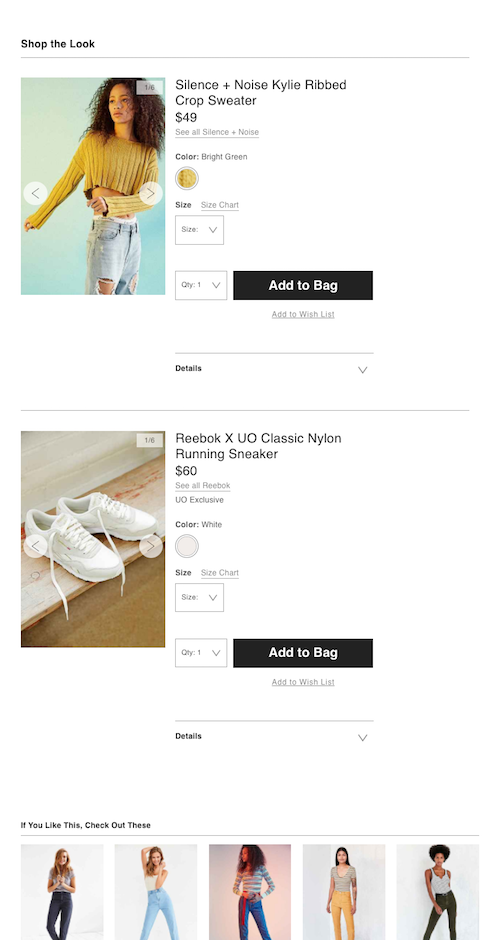A detailed image description for an online shopping platform:

**Screenshot Overview:**
The screenshot features an interface from an online shopping platform showcasing various clothing items and details.

**Primary Item - Crop Sweater:**
- **Title:** Silence + Noise Kylie Ribbed Crop Sweater
- **Price:** $49
- **Description:** The sweater is shown in a perceived mustard yellow color (labeled as bright green), featuring a ribbed texture. It is modeled by a black woman with long, curly, permed hair, who is wearing jeans with torn knees. The crop top falls just below her bust, revealing her midriff. She is looking off to the left.
- **Interface Options:** 
  - Size chart available.
  - Size not selected.
  - Quantity selected: 1.
  - Buttons: "Add to Bag" (black bar with white lettering) and "Add to Wish List."
  - Further product details are accessible at the bottom.

**Secondary Item - Sneakers:**
- **Title:** Reebok EXUO Classic Nylon Running Sneakers
- **Price:** $60
- **Description:** The sneakers are displayed in white, positioned on a stair. Labeled as exclusive.
- **Interface Options:**
  - Size not selected.
  - Quantity selected: 1.
  - Buttons: "Add to Bag."
  - Further product details are available at the bottom.

**Additional Section:**
- **Diverse Models:** The platform shows images of five women (two redheads, one Asian, and two black women), all modeling different outfits. The clothing ranges from black jeans, blue jeans, halter tops, to running wear. 
- **Poses:** Some models are in provocative poses, while others are not.

Everything is set against a white background with black lettering for readability, maintaining a clean and organized interface.